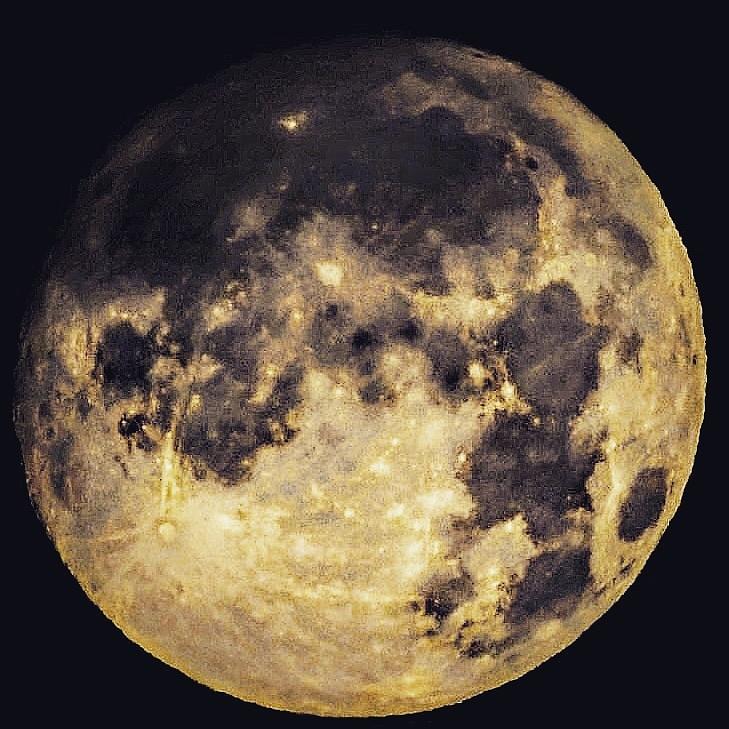This is a detailed close-up picture of the moon, prominently displayed against a black background that makes the celestial body pop. The image, almost occupying the entire frame, provides a high-resolution view of the moon's craggy surface, showcasing numerous craters and divots that underscore its uneven texture. The moon is depicted in hues of gold, with varying shades of brown, gray, and black scattered across its terrain. Lighter tones of gold and summer-brown color the brighter areas, adding depth and contrast. Notably, the moon's upper left section appears darker, while the lower right is brightly illuminated, likely reflecting the angle of sunlight. Interesting striations and lines radiate from a distinct rounded spot, reminiscent of a watermelon top. The overall interplay of light and shadows across the surface, along with the detailed craters and reflective spots, creates a visually captivating and scientifically intriguing portrayal of our lunar companion.